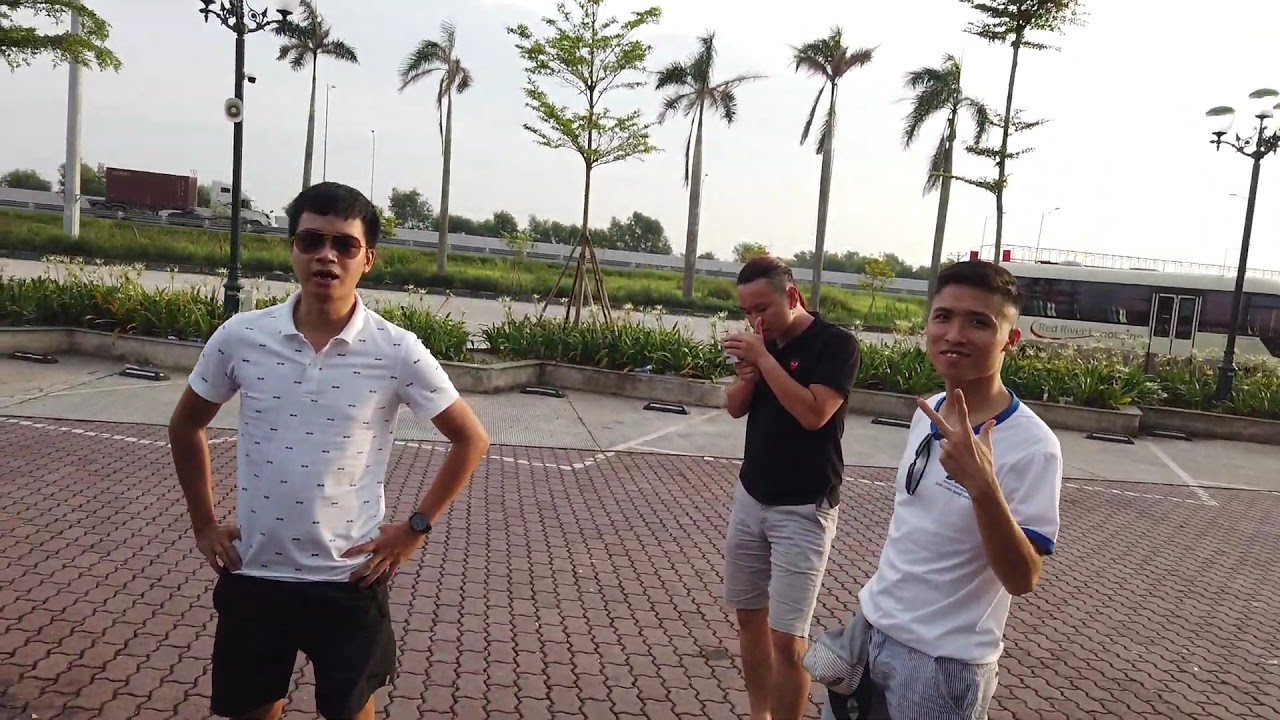In this outdoor photograph, three young men are captured on a paved walking path adorned with brown tiles and flanked by plants in pots and lush greenery. The man on the left, wearing sunglasses, a white t-shirt, and black shorts, stands with his hands on his hips and gazes confidently at the camera. The man in the middle, distinguished by his black t-shirt and grey trousers, is focused on lighting a cigarette, with his head slightly tilted downwards. On the right, a cheerful man in a white t-shirt holds up a victory sign while smiling directly at the camera. The backdrop features vibrant palm trees and colorful flowers, suggesting a tropical climate possibly in Southeast Asia. In the distance, a road is visible with a moving truck and a stationary bus adding a hint of urban life. The sky is clear but appears white, indicating a bright, hot day. The overall scene is a candid yet warm depiction of friends casually enjoying a moment together.